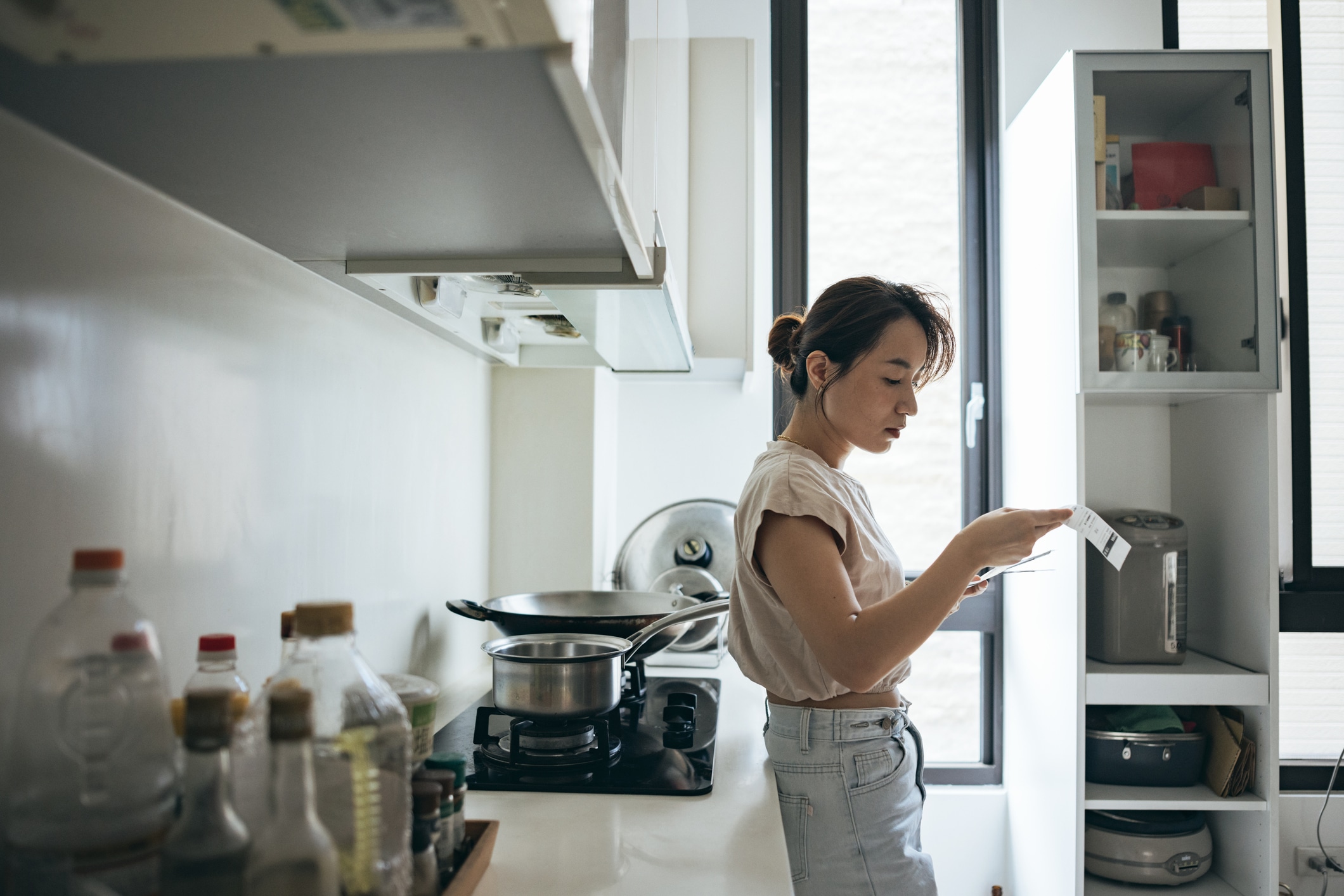A young woman stands in a well-lit, modern kitchen, the space illuminated predominantly by natural daylight. She is positioned with her back against a white or off-white stone countertop, which features an assortment of bottles—likely olive oil, cooking oil, vinegar, and spices. The kitchen has a sleek, black gas stovetop on which a wok and a handled pan are placed, both lids set aside on what appears to be a drying rack by a nearby window. Above the stove, an extraction fan and light fixture blend subtly into the scene, unlit amidst the ample daylight.

The woman, attired in light-colored jeans that almost appear white and an untucked, sleeveless t-shirt exposing a hint of her midriff, holds a stack of papers, her dark hair gathered into a ponytail. To the right, an open cupboard reveals various kitchen items. The top shelves, encased in glass doors, are stocked with spices and other cooking essentials. Below, a larger middle section possibly contains a rice cooker, along with more kitchen gadgets and utensils stored in the shelves beneath.